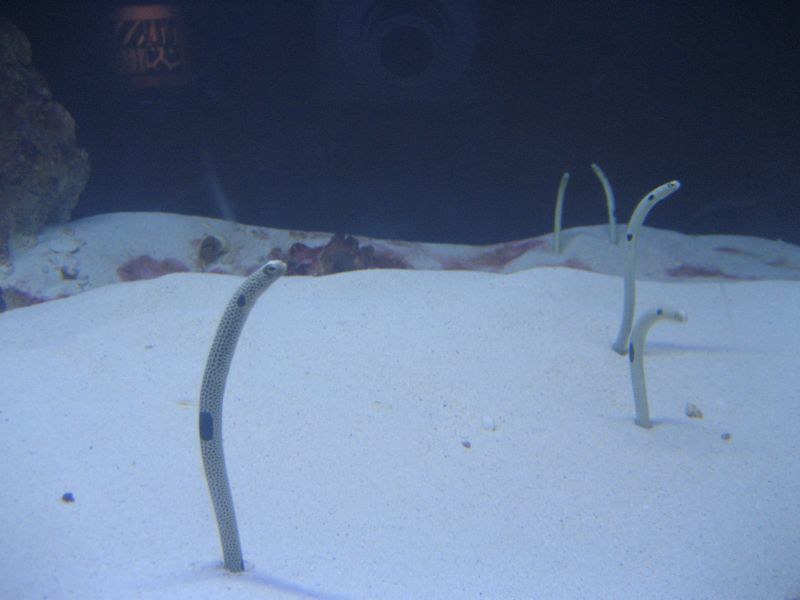The photograph captures an underwater scene, possibly taken in an aquarium or ocean, showcasing a seabed covered with fine white sand and small rocks. Emerging from the sand are several thin, worm-like creatures adorned with blue and white spots, each featuring a distinct eye and larger black oval markings on their bodies. Some of these creatures are sticking straight up, with others bent over in various directions. Toward the left of the image, one of these creatures is prominently visible, while a few others can be seen on the right and in the background. The lighting, likely from the photographer, casts a unique glow on the scene, giving the white sand and blue background a somewhat surreal appearance. Additionally, the left side of the photograph features an illuminated object with zebra-like stripes, adding a touch of mystery to the overall scene.